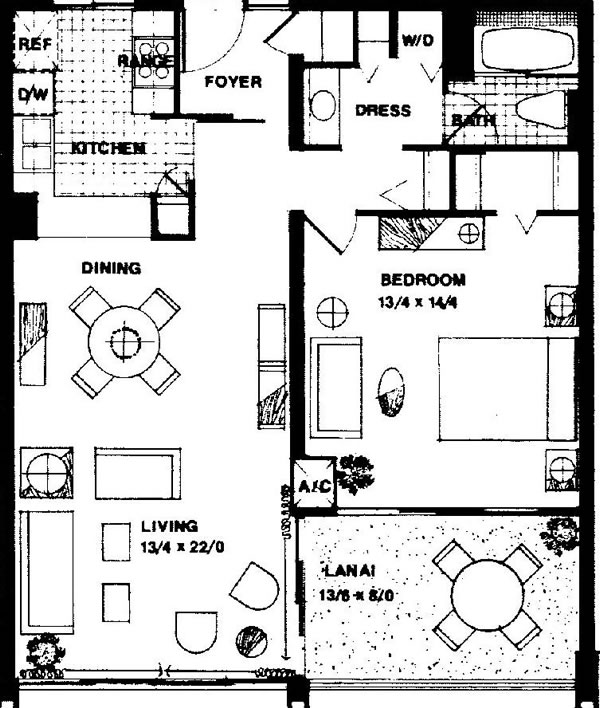The image illustrates a basic rectangular floor plan of a house. The entrance to the house is located on the north side. Upon entering, you are greeted by a foyer. To the right of the foyer is the kitchen. Moving past the kitchen, you enter the dining room, which seamlessly flows into the living room due to the open floor plan design that combines these two areas. The layout also includes a bedroom that measures 3 by 14 square feet, situated along the south side of the house. Directly opposite the bedroom is a bathroom. The living room grants access to a patio, which is an additional feature of the house.